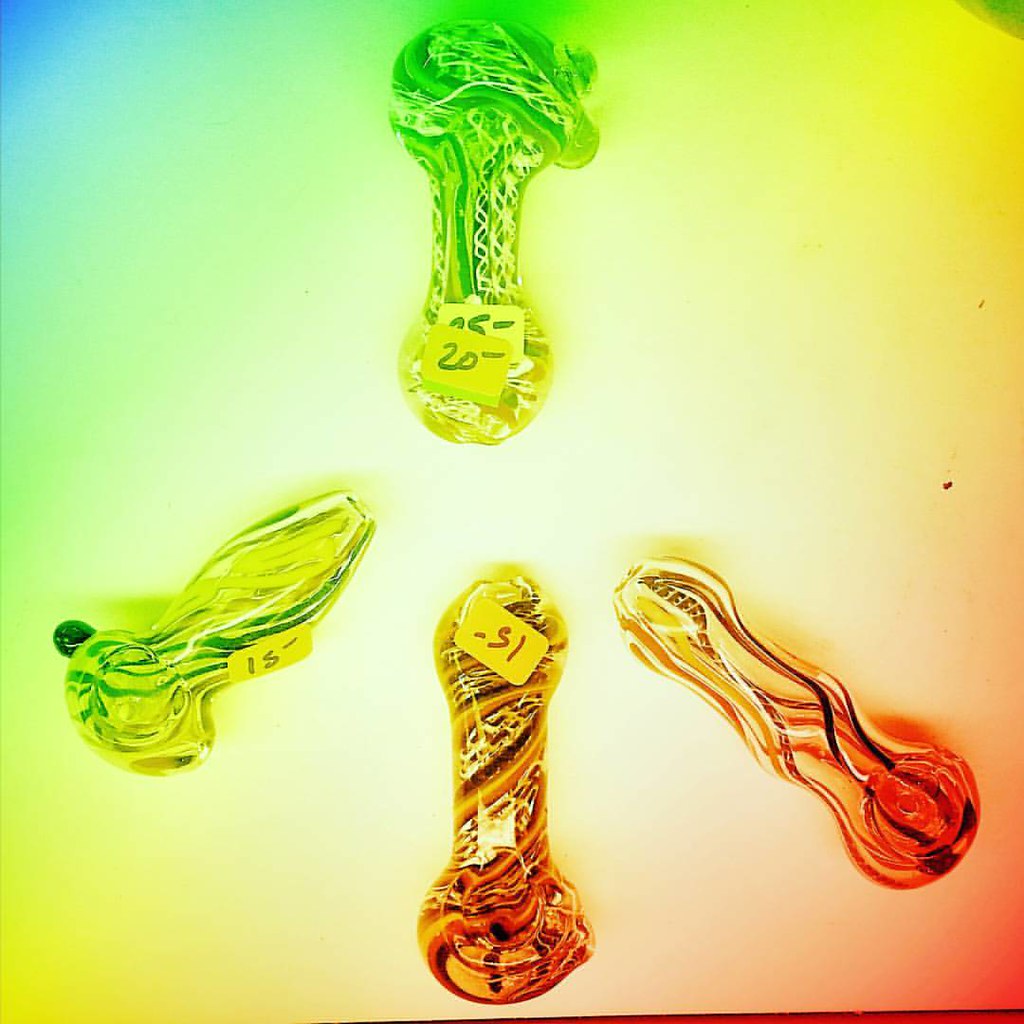The image features a vividly illuminated rainbow background transitioning from blue to green, yellow, orange, and red, with intense lighting enhancing its brightness. Centrally positioned are four intricately designed glass smoking pipes, commonly used for smoking marijuana or tobacco. These pipes exhibit colorful swirly patterns and artistic glass bubbles. Arranged in a semi-circle with one at the top and three at the bottom, the pipes vary in color and design. The top pipe sports a price tag of $20, while the bottom left and center pipes are marked $15 each. The bottom right pipe lacks a price tag. Despite the vibrant filter distorting the true colors, the distinct rainbow overtones add a mesmerizing, almost surreal quality to the image.